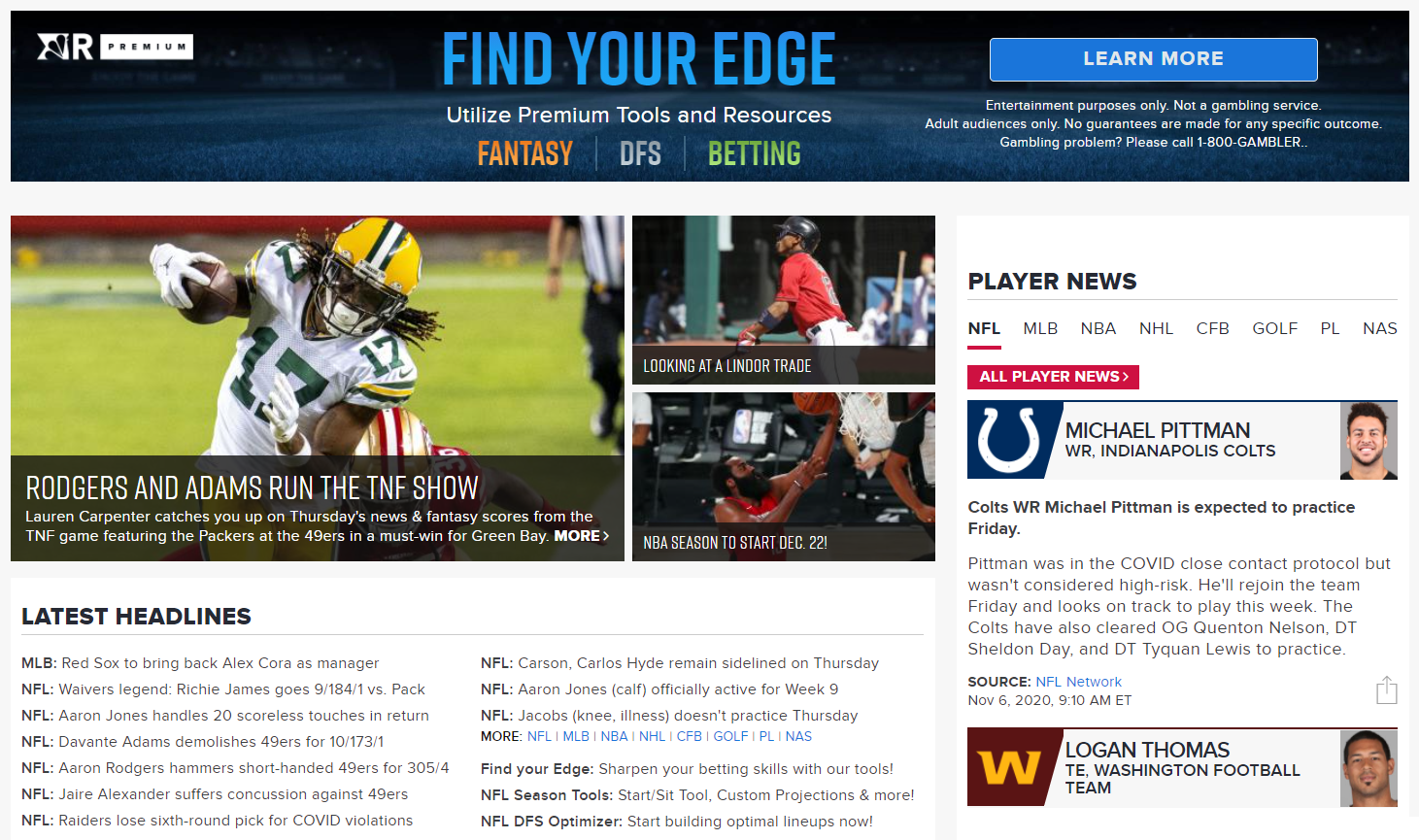This screenshot captures a vibrant sports-themed website. At the top of the page, an "R" symbol with a premium logo marks the branding. In bold blue text, a banner reads, "Find Your Edge. Utilize premium tools and resources," followed by options for Fantasy, DFS, and Betting. To the right, a blue "Learn More" button stands out. Below, a disclaimer states: "Entertainment purposes only. Not a gambling service. Adult audiences only. No guarantees are made for any specific outcome. Gambling problem? Please call 1-800-GAMBLER."

A dynamic image of a football player dominates the screen. The player wears a white jersey featuring green number "17" and a green and yellow stripe on the sleeve. A yellow helmet with a central black stripe partially conceals his long braids or dreads, which fly outward as he runs with the football. The player is clearly in motion, intensifying the action-oriented theme of the site. A referee is visible in the corner of the picture.

Adjacent to this main image, two additional sports-related pictures provide more visual interest. To the far right, a column titled "Player News" lists abbreviations for various sports leagues, including NFL, MLB, NBA, NHL, CFB, Golf, PL, and NAS. Highlighted at the bottom is a headline about Michael Pittman, Wide Receiver for the Indianapolis Colts.